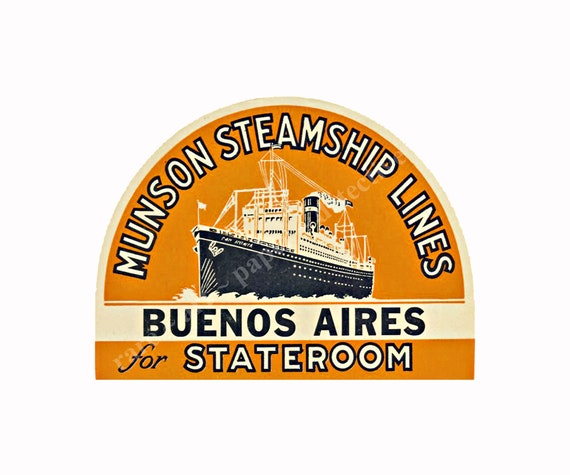This image appears to be a vintage advertisement or label, possibly designed as a sticker or a patch, for Munson Steamship Lines. It has a distinctive cathedral shape with a half-circle at the top and a straight line at the bottom, bordered in beige with an orange interior background. The top of the label features the text "Munson Steamship Lines" in white. 

Below the text, a large, vintage steamship is prominently depicted. The steamship has a black hull adorned with rows of windows, and an upper structure in white with multiple levels and additional windows. At the front of the ship, a white flag is visible, and steam can be seen billowing from a large chimney at the back, indicating the ship is in motion. The hull of the ship cuts through the water, creating splashes at the bottom of the image.

Underneath the steamship, "Buenos Aires" is printed in black text on the beige background. Further below, there’s an orange rectangle containing the phrase “For State Room” in white cursive text with a black background trimming. A difficult-to-read watermark spans from the bottom left to the top right across the design, adding to the vintage feel of the label.